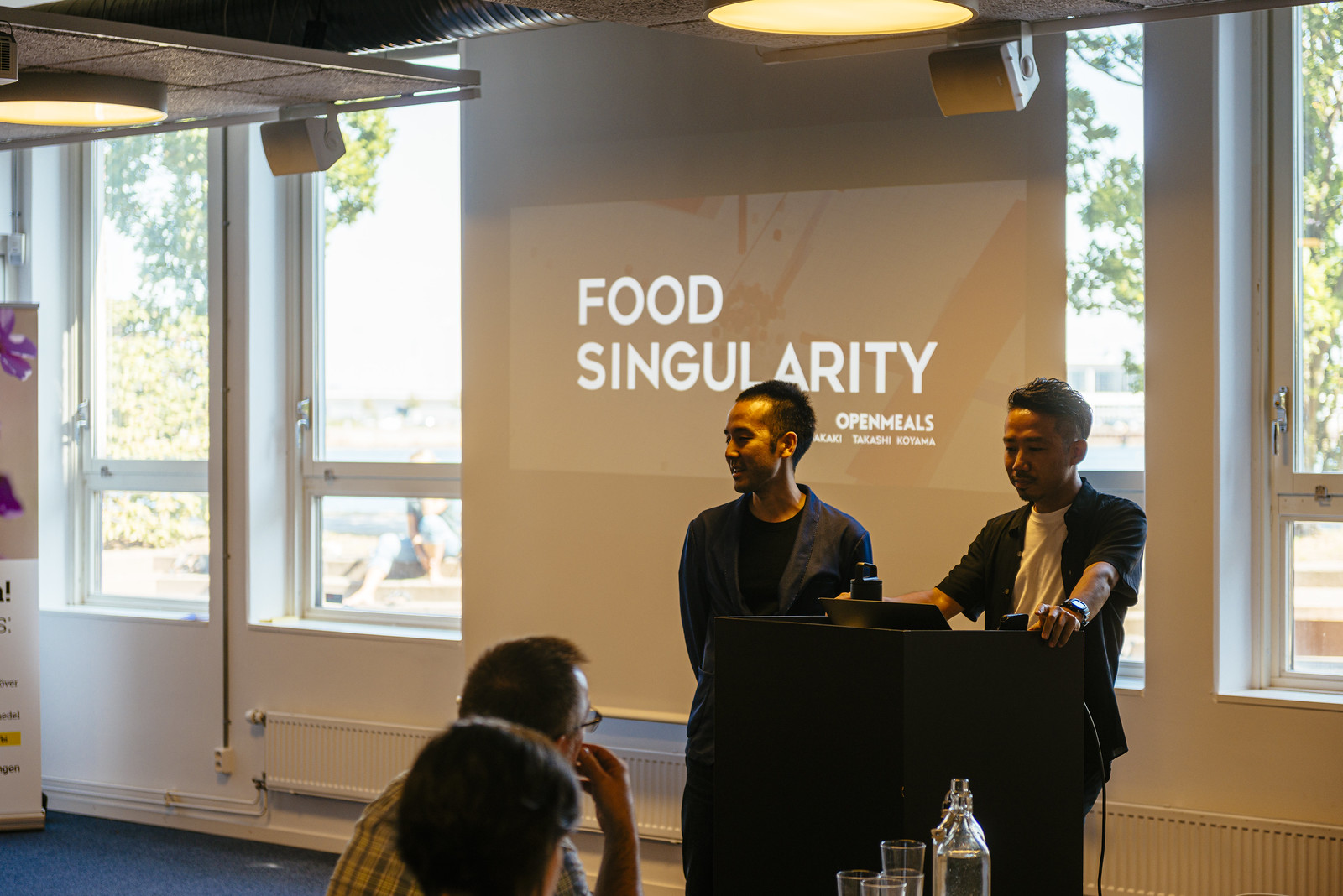This photograph captures two Japanese men standing behind a dark-clothed podium, seemingly giving a speech or holding a presentation. Both men, who have short black hair, are dressed in black blazers, with one wearing a black t-shirt and the other a white t-shirt underneath. One man is focused on the podium, arms outstretched as if preparing to read, while the other looks towards the audience. In the foreground, the backs of two heads—a man and a woman—are visible, seated at a table with several cups and a bottle of water. The man has glasses, a yellow dress shirt, and his right hand raised to his mouth, appearing thoughtful. Behind the presenters is a long white wall with numerous rectangular windows, allowing bright sunlight to filter through. A projector screen hangs in front of some windows, displaying a slide that reads “Food Singularity” with “Open Meals” and the name Takashi Koyama at the bottom.